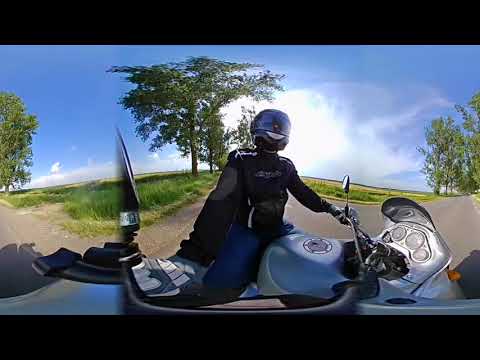The image depicts a person fully clad in motorcycle gear, riding a silver and light blue motorcycle on an open country road. The individual, whose gender is indistinguishable, is wearing a black helmet with the visor down, a black driving suit covering them from head to wrists, silver gloves, and blue pants. The road is devoid of other vehicles and appears to be made of asphalt, flanked by green grass and a few trees. Above, the blue sky is dotted with a few wispy white clouds, with the bright sun sitting just above the horizon. The motorcycle, with intricate details including three indicators on the right, is positioned to the right side of the image. The composition includes horizontal black stripes at the top and bottom, framing the vertically-oriented photograph.